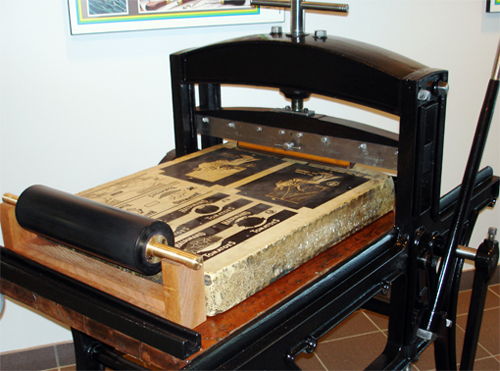This image depicts an antique rolling or printing press machine with a predominantly black frame. At the center of the device is a large wooden piece that appears to have some kind of faded writing on it, though the text cannot be clearly discerned. Its top features a rounded wooden arch with a central silver rod that includes a handle for adjusting the machine. Below this arch are silver bolts and an orange-lined blade. 

The press also has a noteworthy base: a combination of what appears to be a wooden table supporting a large, light cream-colored stone slab, adorned with black text and drawings. On the base's left side, a black cylindrical roller with gold arms is situated, indicative of its role in the printing process. The background reveals a white wall with the edge of a picture frame and a partially visible image, alongside a brown-tiled floor.